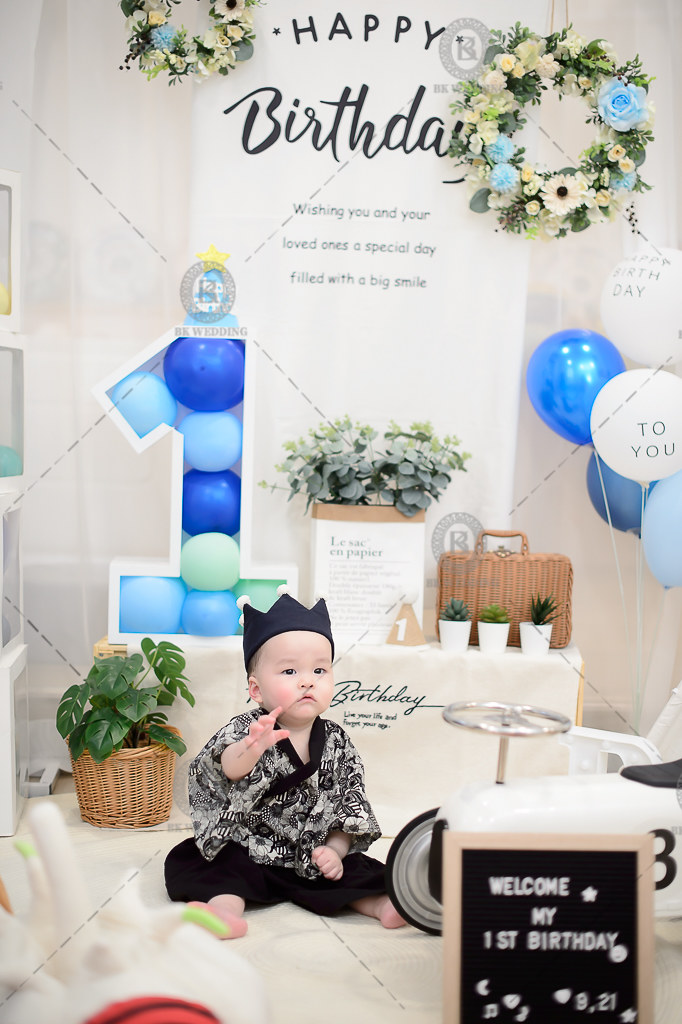A vividly detailed photograph captures a young Asian boy celebrating his first birthday, adorned with a felt black crown featuring white plush balls on the points. The little boy, dressed in a black and white kimono with matching pants, sits on a white platform draped with fabric, giving the appearance of a bed or table. In front of him stands a black and white old-fashioned race car and a chalkboard sign reading, "Welcome to my first birthday."

The scene is adorned for the festive occasion, with a small table behind the boy covered in a white tablecloth that says "Birthday," followed by the phrase "Live your life and forget your age." Atop the table rests an array of decorations: a large number one filled with blue, white, and dark blue balloons, a suitcase, and three small plants in white buckets. Additionally, blue and white balloons are arranged to the right side of the composition.

The backdrop features a large white poster with the words "Happy Birthday" in bold black text and the heartfelt message, "Wishing you and your loved ones a special day filled with a big smile." This poster is flanked by two green flower wreaths with white and blue blooms. A wicker basket with more green plants adds to the charming and homey decor. The entire setting is a joyful celebration of the boy's milestone, brought to life with meticulous details and festive decorations.